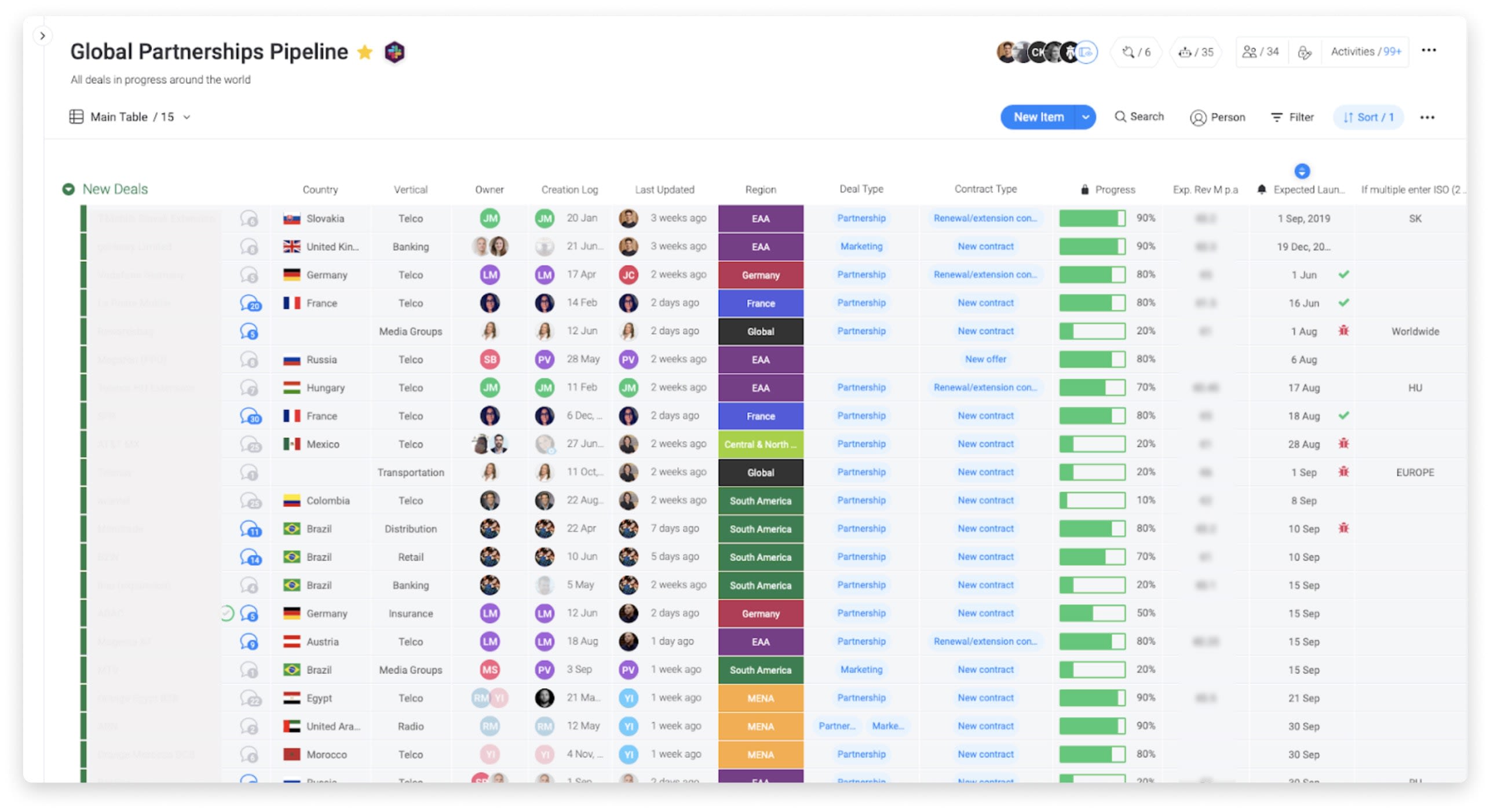This image showcases the "Global Partners Pipeline" interface, with the title prominently displayed in bold black text. To the left of the title, there's a yellow star icon and a hexagon segmented into red, blue, green, and yellow sections. Below the title, a central table is visible, with "15" indicated alongside a drop-down menu. On the right side of the interface, a series of profile pictures is displayed next to various icons and buttons. These include a forward slash icon, a "plug" symbol, another forward slash, with associated numbers like "6," "35," "33," and an activities count labeled "99+."

A prominent new item button appears in blue with a pull-down menu, accompanied by search, filter, and sort options, all in lighter blue. The main portion of the screen resembles a database with headers for columns such as "New Deals," "Country," "Vertical Owner," "Creation Log," "Last Updated," "Region," "Deal Type," "Contract Type," "Progress," "EXPREVMPA," "Expected Launch," and a note for multiple entries, "ISO (2)..."

The table is densely populated with entries, which fill the page, and some entries are highlighted in green. Overall, the interface appears to be a comprehensive dashboard for managing ongoing global deals and activities.